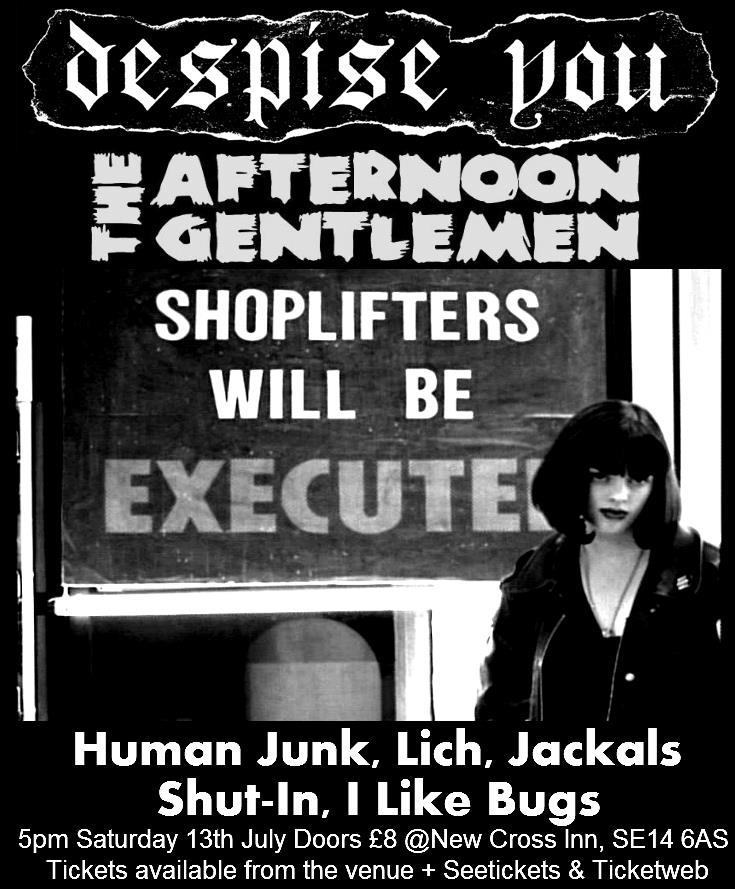The black-and-white poster features a grungy collage-style design with prominent white text at the top that reads "Despise You," as if it has been cut out from another magazine, adding a raw, torn-edge effect and visible wrinkle marks. Below this, in smaller white text, it reads "The Afternoon Gentleman." A central image depicts a stern-looking white woman with chin-length straight black hair, black lipstick, wearing a black jacket and a necklace, positioned next to a sign that says "Shoplifters Will Be Executed." She exudes an edgy, defiant attitude. Beneath the image, the poster lists several band names in large white font: "Human Junk," "Litch," "Jackals," "Shut In," and "I Like Bugs." The poster details the event taking place at 5 p.m. on Saturday, 13th July at New Cross Inn, SE14 6AS, with doors opening at 8 quid. Tickets are available from the venue, See Tickets, and TicketWeb.